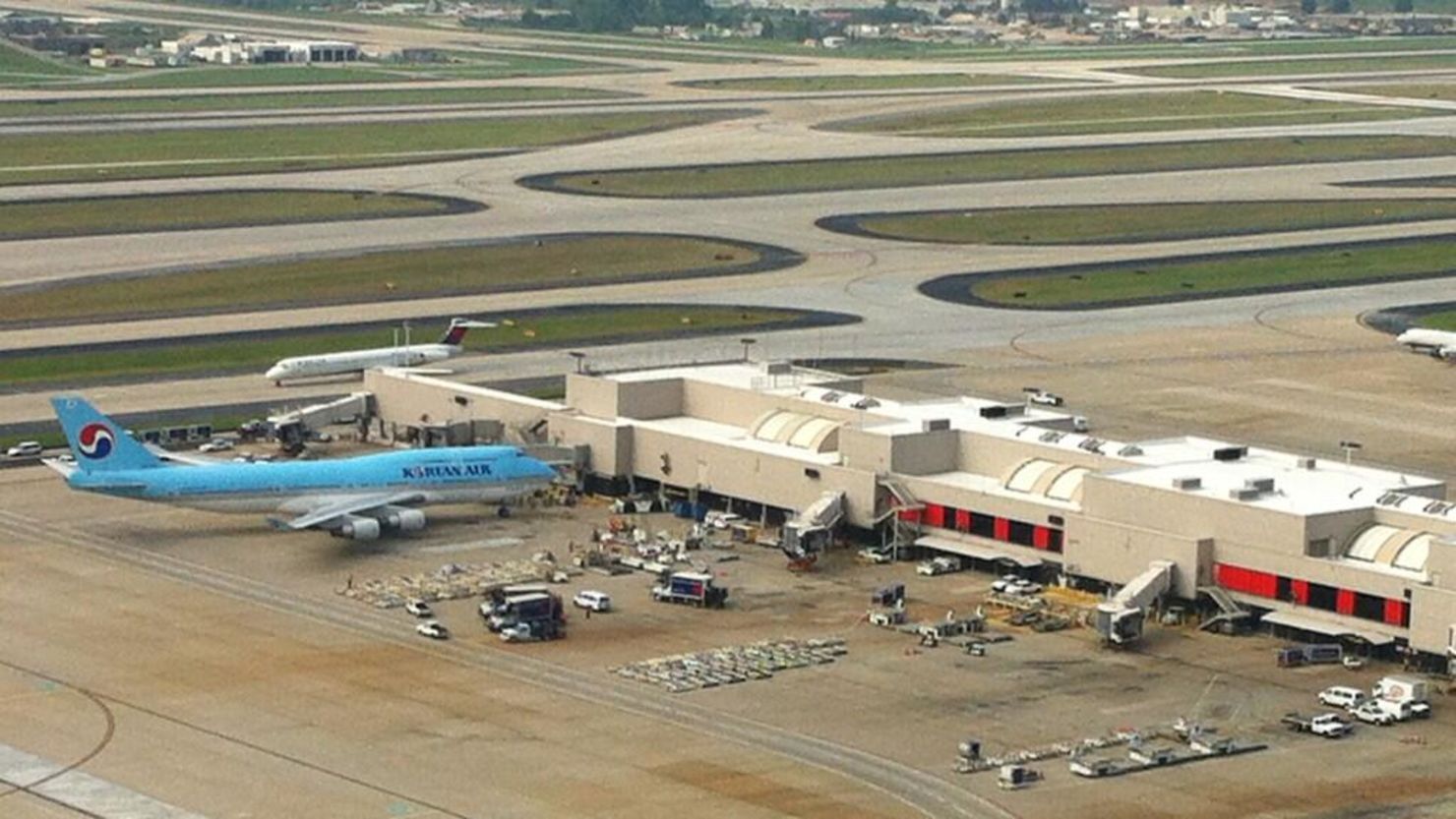This elevated photograph of an airport precinct prominently features a cream-colored airline terminal at the center. The terminal has extensions for passenger access to planes, with red-framed windows and a white roof. Stationed at one of the gates to the upper left of the terminal is a large light blue Korean Air airplane, which boasts a red, white, and blue insignia on the tail and the airline's name in black letters on the fuselage. To the immediate left of the Korean Air plane is a smaller white aircraft with a blue and red tail.

The foreground of the image is bustling with activity, as numerous luggage carriers, maintenance carts, trucks, and vans are scattered around. Notably, a plane's nose is visible coming from the center right. Spanning from the left side to the background, the ground is flat and brown, with several interconnected runways and taxiways separated by green grass strips. There are no planes currently using the runways. Finally, in the far distance beyond the airfield and runways, there are buildings that resemble houses or businesses, providing a backdrop to the busy airport scene.